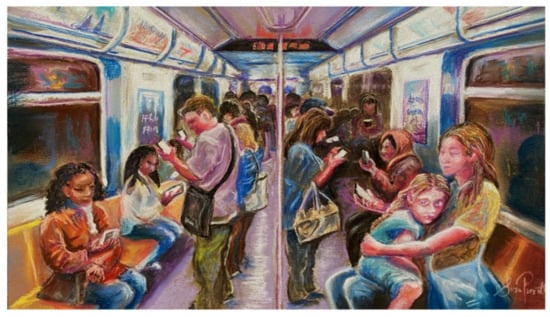This detailed painting vividly captures the bustling interior of a subway train, portraying the diverse array of passengers engrossed in their daily activities. Central to the composition, a young woman in a yellow shirt sits near the front right, with a small child in a blue shirt perched on her lap, gazing out towards the viewer. Behind her, an elderly woman wearing a babushka headscarf interacts with another seated woman dressed in a blue shirt and gray pants who clutches a purse. The scene is enriched by the detailed depiction of the subway bar running vertically along the car, a common feature for passengers to hold onto. 

To the left, a multiethnic cast of characters continues to fill the train. A person clad in a purplish shirt and greenish pants stands close by, absorbed in their phone, their black satchel hanging at their side. Further left, two women sit in the typical orange subway seats: one in an orange jacket and blue jeans, the other in a white shirt and blue jeans. Among them, touching details include the young lady in a red coat with curly hair, also deeply absorbed in her phone, and across from her, an elderly woman similarly engaged.

Standing passengers, meticulously illustrated, include a man positioned centrally in the aisle with a black messenger bag over his shoulder, seemingly engrossed in reading something on his phone, mirroring the focused demeanor of another woman nearby. A notable detail includes a young woman at the bottom right, with a distinctive blue carrier bag slung over her arm, highlighting the universal prevalence of digital devices in modern commuting life. The painting is signed at the bottom right, though the artist's name remains indecipherable. This rich tableau offers a snapshot of urban life, blending individual stories in a communal space.